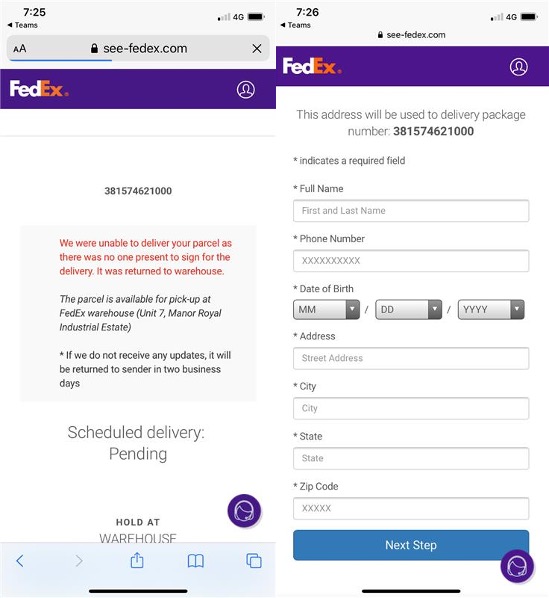Two side-by-side screenshots from the FedEx mobile site in Safari depict a delivery issue. The left screenshot shows a message stating, "We were unable to deliver your parcel as there was no one present to sign for the delivery. The parcel is available for pickup at the FedEx warehouse," followed by an address. It includes a delivery package number and an option to schedule a redelivery or request a hold at the warehouse. The right screenshot, accessed by clicking a link on the left, instructs the user to input their full name, phone number, date of birth, and other details to redirect the delivery. A "Next Step" button is at the bottom, suggesting continuation of the redirection process.